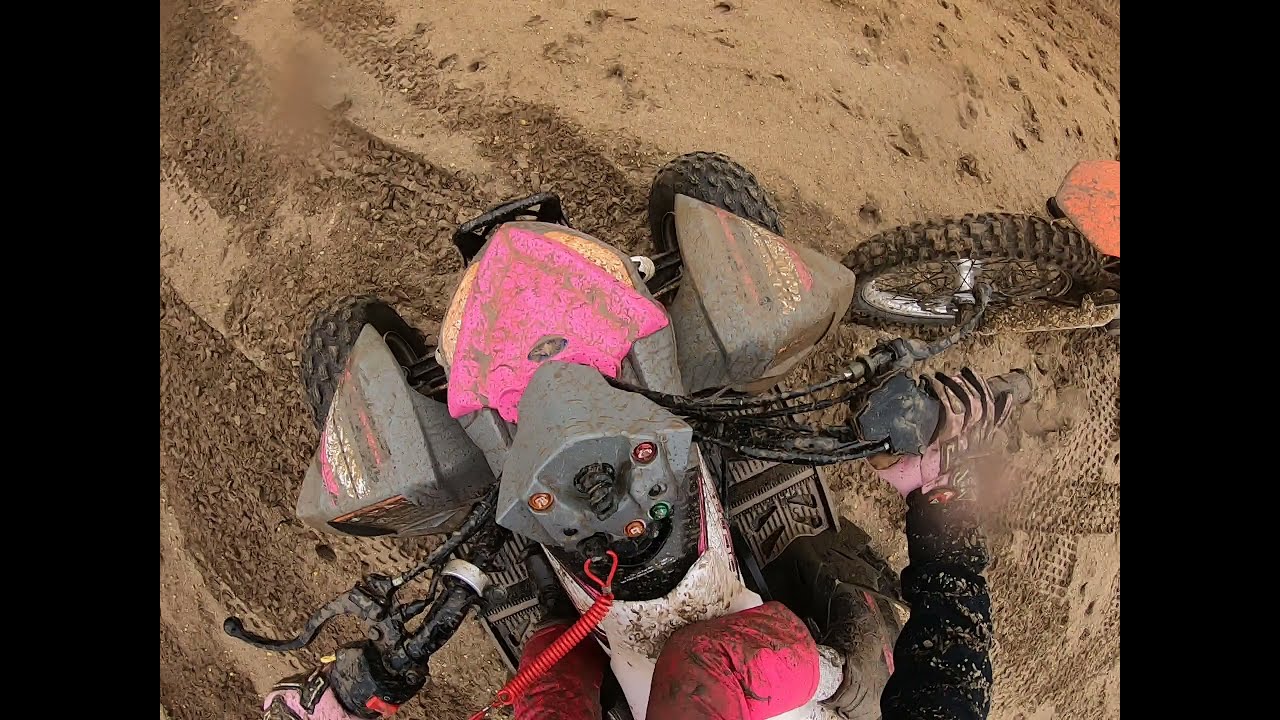The image is a top-down perspective photograph, depicting a person riding a bulky, four-wheeled ATV through a muddy, dirt-covered terrain. The ATV is primarily pink and gray, with a distinct pink triangle on the hood. The rider's arms, clad in a black-sleeved jacket and pink gloves, are visible gripping the handlebars, while their red pants add a splash of color. To the right side of the image, partially obscured, is another dirt bike with an orange wheel, seemingly contributing to the dirt flying through the air. The ground is a mix of dark and light brown mud, thoroughly churned by previous rides, accentuating the motion and ruggedness of the scene. Vertical black bars frame the left and right sides of the image.